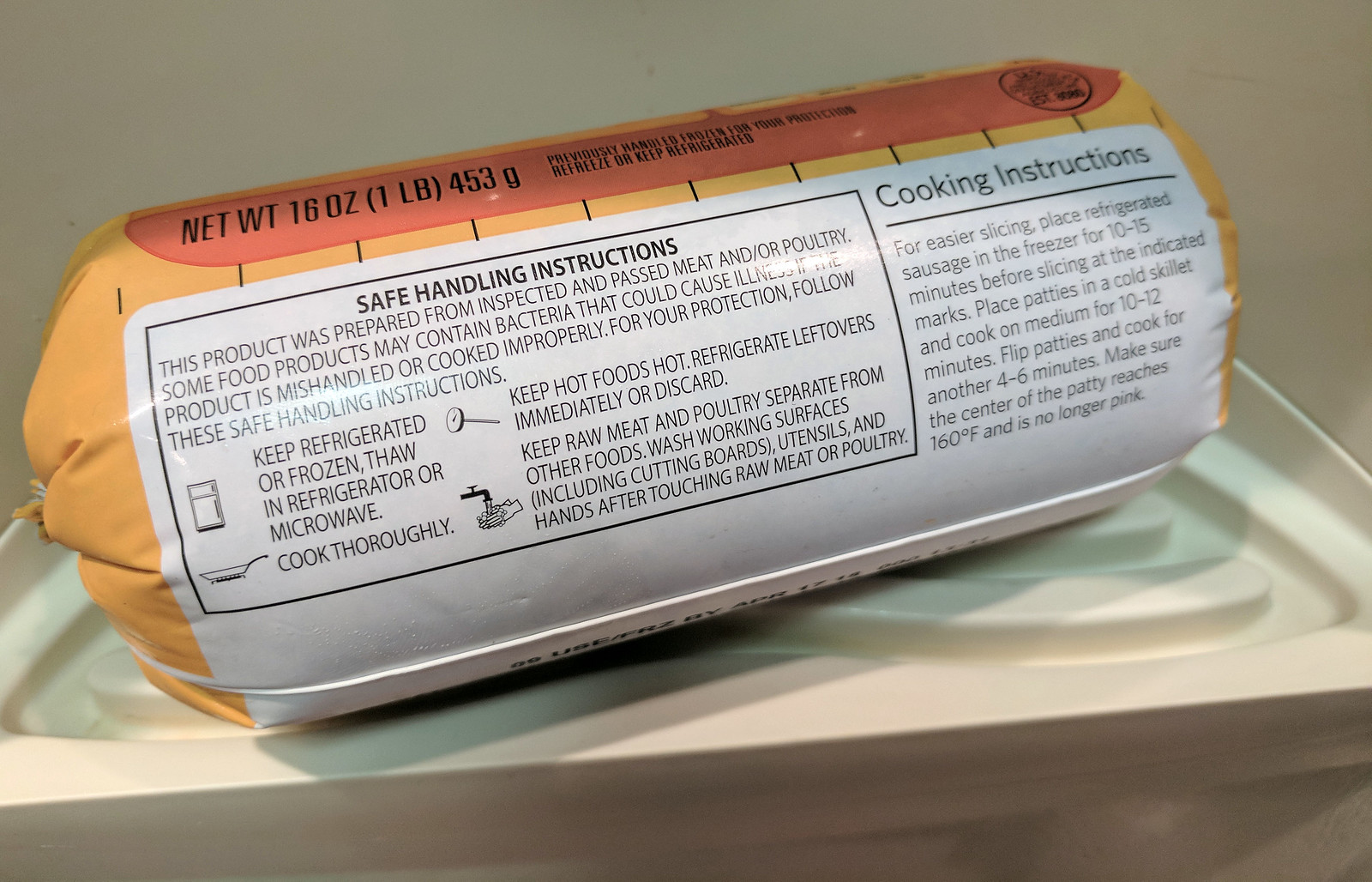This photograph captures a packaged sausage placed on an off-white plastic tray. The package is positioned horizontally, slightly tilted with the lower left closer to the viewer and the upper right oriented further away. The top of the packaging features a dark brown band with black text indicating the net weight, "16 oz (1 lb) 453 grams," alongside additional text and a logo. The central portion of the packaging is a light brown, orangey hue, mostly obscured by a prominent white, rectangular label with rounded corners. This label covers the majority of the sausage package and includes "Safe Handling Instructions" in a boxed section with a black border and heading. To the right of this section, another heading reads "Cooking Instructions," underlined in black, followed by detailed cooking guidelines.